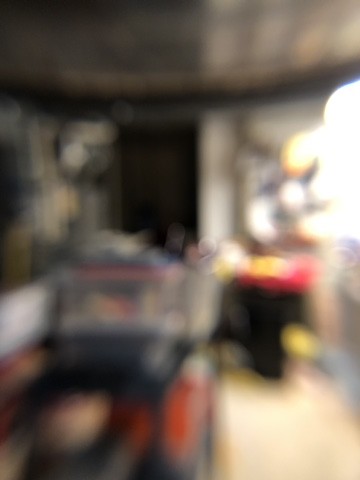A highly blurred and unfocused indoor image featuring a chaotic blend of colors. On the right-hand side, there appears to be an intensely bright white area, likely a window providing light from the outside. Dominating the foreground is a black rectangular object with a gray or silver section on top, adorned by a red button on the right and several indistinct color patches on the front, including salmon, dull red, and gray hues. Further into the image sits another black object topped with red, featuring yellow elements both at its top and midway down its side. Across the upper portion of the image, about one-fifth from the top, is a brown, arch-like structure stretching horizontally across the frame. Behind this structure lies a dark rectangular shape, possibly a door. The composition and its components are ambiguous, leaving the purpose or subject of the photograph unclear.